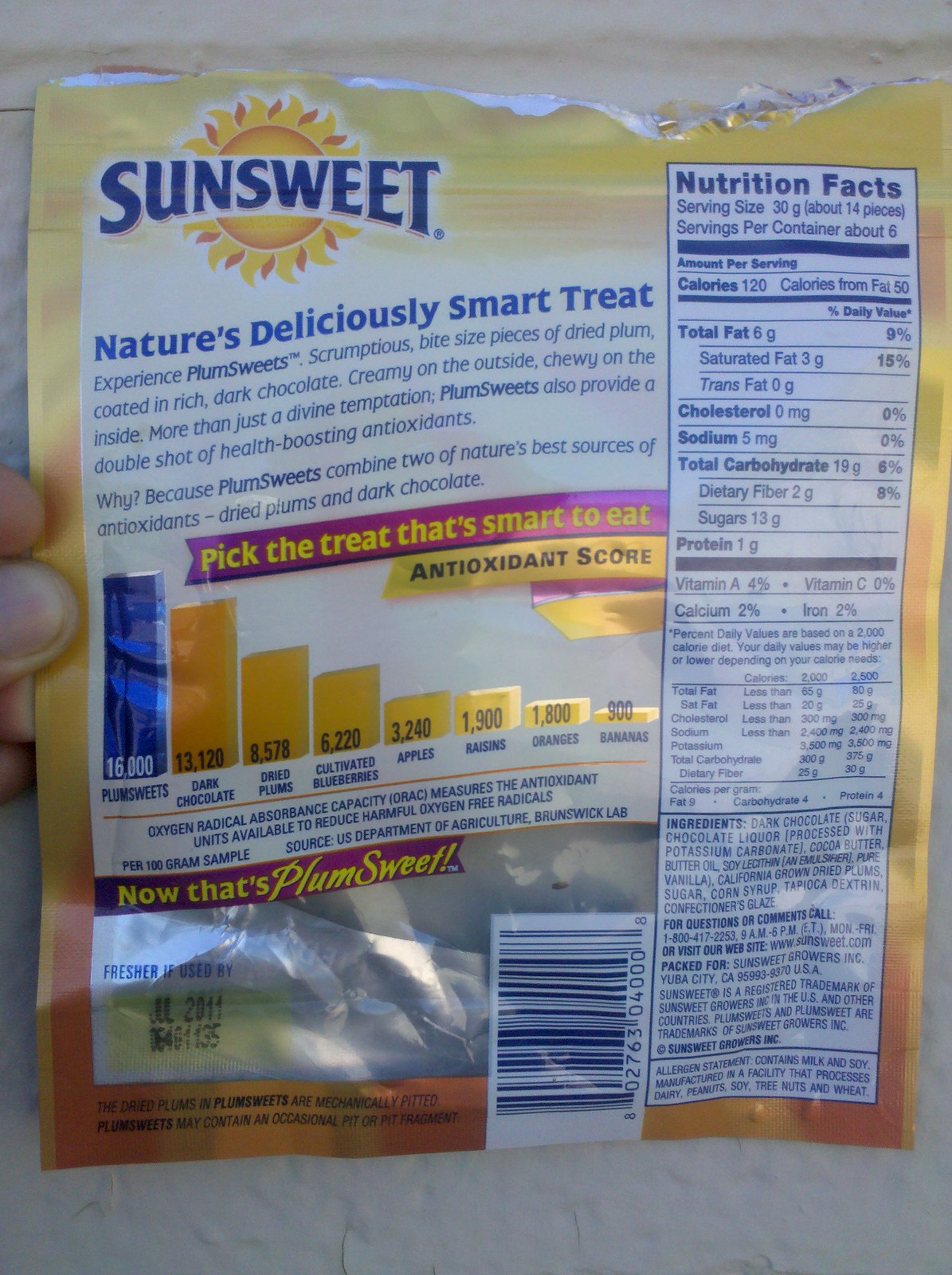This close-up image captures the back of a SunSweets Plumsweet package, prominently featuring a mix of detailed information and colorful graphics. On the right side, a large rectangle outlined in blue displays the nutrition facts in blue text, detailing serving size (about 14 pieces), servings per container (about 6), calorie count, total fat, cholesterol, sodium, total carbohydrates, and protein content, along with details on vitamins A and D, calcium, and iron. Below this section, the ingredients list and a contact number for inquiries are provided.

On the left side, the top shows the SunSweets logo in blue text, set against a yellow sun silhouette with radiating orange and yellow flames. Beneath the logo is the tagline "Nature's Deliciously Smart Treat," followed by two paragraphs of descriptive blue text extolling the health benefits of the product. Below this text, a color-coded chart displays antioxidant scores, with a tall blue line next to descending orange lines, comparing Plumsweet to other fruits like apples and bananas.

Additional details include a white top background with jagged edges indicating the package has been ripped open, a thin gold border around the package, and a silver area at the bottom left showing the expiration date, adjacent to a QR code. A piece of finger can be seen holding the package from the left side, with a thumb extending onto the side, emphasizing the human interaction with the package.